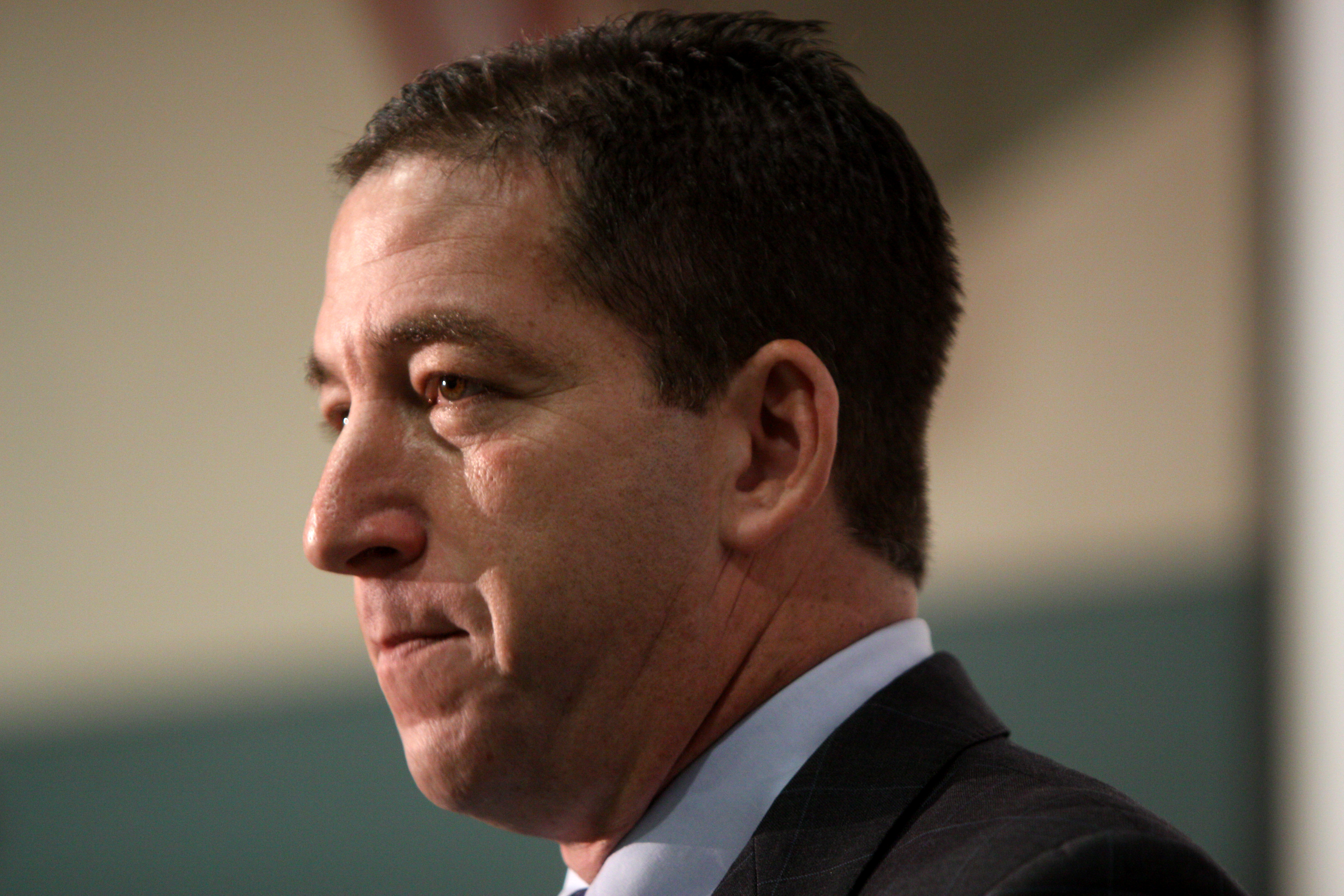This side-profile photograph captures a man from the shoulders up, centered in the frame within an indoor setting. The background features a white wall on the top half and a turquoise blue band on the bottom half, though it appears out of focus due to the emphasis on the man. A white support beam is visible on the right side of the image. The man is looking towards the left, dressed in a black business coat over a light blue button-up shirt with the collar turned down. He has short brown hair and brown eyes, and his expression conveys a sense of determination or grimace, with lips slightly pursed. Ambient lighting from the left highlights his face, accentuating his contemplative and resolute demeanor.